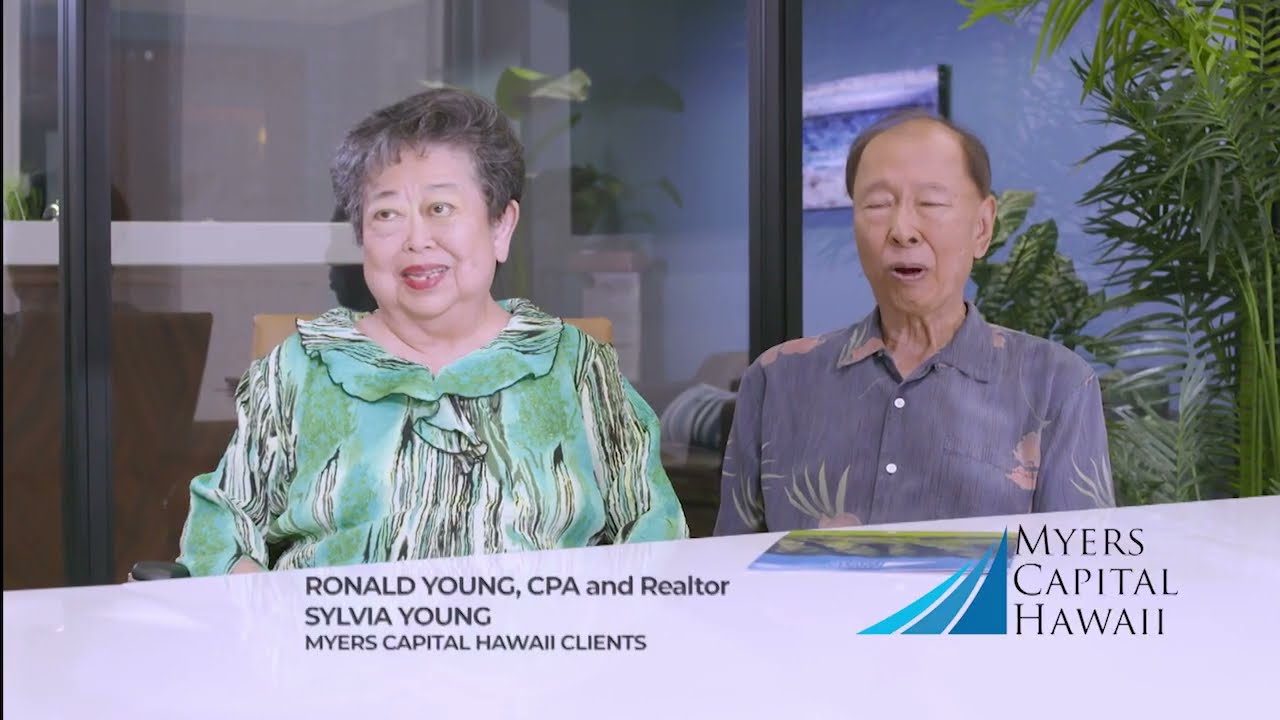This image appears to be a screenshot from a video or TV show, likely an advertisement for a real estate investment company, possibly Myers Capital Hawaii. The setting is an indoor office space with blue walls, featuring a large glass window in the background. Through the window, a couch and a blue painting are visible, creating a relaxed, professional ambiance. In the foreground, two Asian individuals are seated: a woman on the left and a man on the right. The woman, identified as Sylvia Young, has short black and gray hair and is wearing a green, white, and black blouse. The man, identified as Ronald Young, is dressed in a gray button-down collared shirt with a brown and white floral print. A very tall green plant is situated to the right, adding a touch of greenery to the scene. Underneath them, a white rectangular stripe displays black text: "Ronald Young, CPA and Realtor" and "Sylvia Young, Myers Capital Hawaii Clients." To the right of this text stripe, in black large letters, it reads "Myers Capital Hawaii," accompanied by a logo with three shades of blue resembling sails on a boat. Ronald's eyes are slightly closed, and it appears he is speaking, suggesting an interview setting.